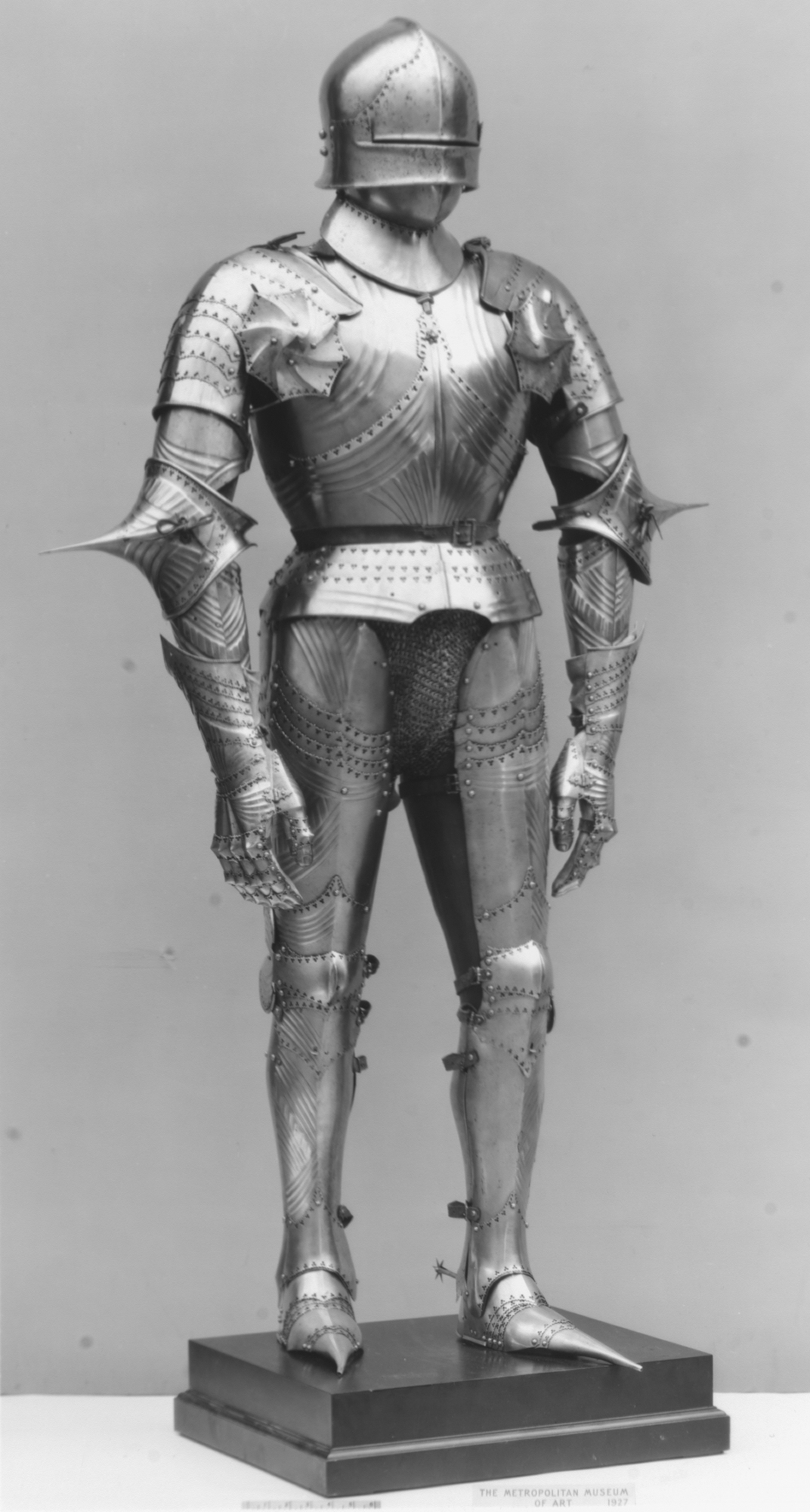This vertical rectangular black-and-white photograph depicts a meticulously crafted suit of medieval knight's armor, arranged for display. The armor, made of shiny silver metal, encases the figure from head to toe, lending it an almost robotic appearance. The knight stands upright on a two-tiered black pedestal against a grayish-blue background. Each piece of the armor, fastened together with rivets, contributes to the overall protective ensemble. The feet are notably covered with pointed metallic toes, and spurs can be seen at the heels. Moving upward, the legs and arms, both armored, feature sharp, pointy attachments at the elbows. The torso is shielded by a segmented chest plate and waist guard, while the helmet, complete with a faceplate, extends down to cover the entire head. This suit of armor would leave little exposed to any potential threat. A faint watermark at the bottom reads "The Metropolitan Museum of Art 1927," subtly indicating its provenance.